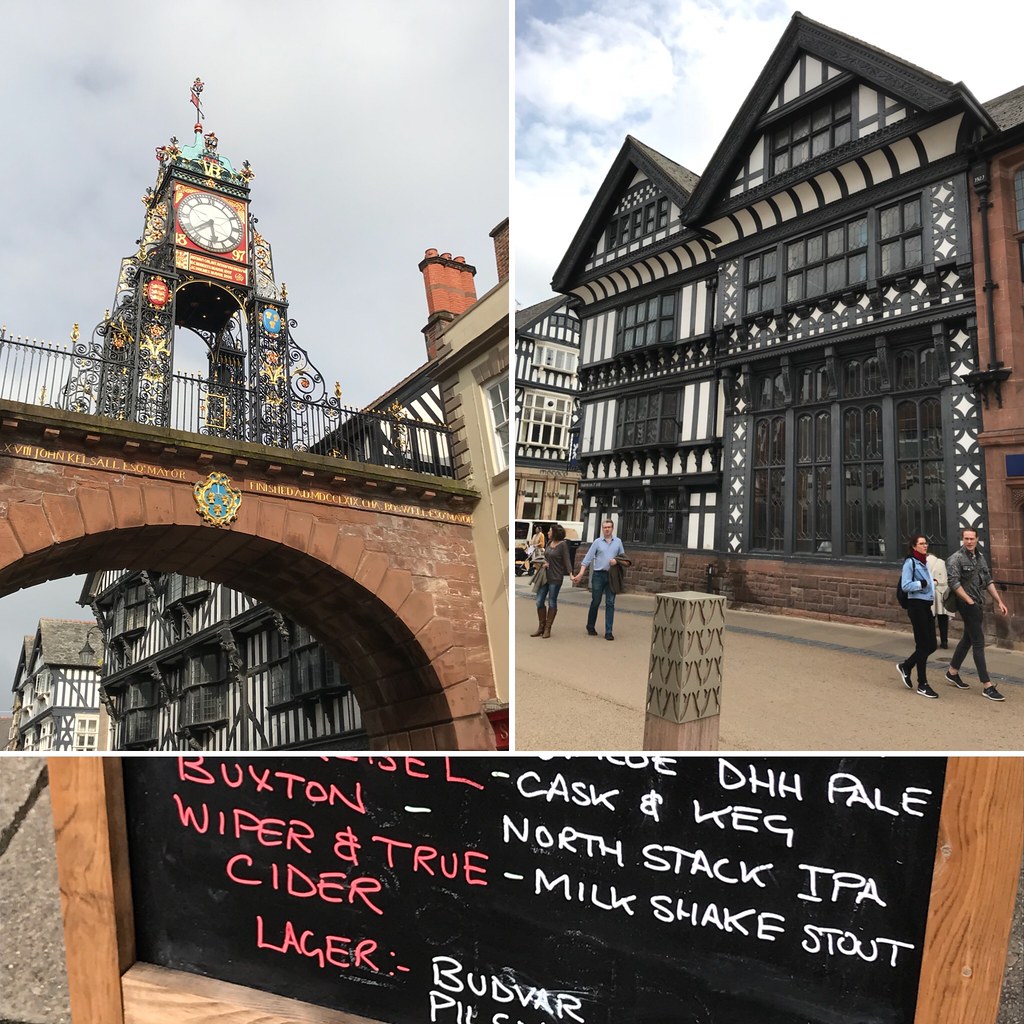The image is a collage featuring two photos on the top and one photo spanning the bottom. The top left photo showcases the historic Eastgate Clock, an ornate landmark in Chester, UK, known for its intricate metal designs and prominent white analog clock atop a sharp-pointed structure. In the upper right, there's an image of Underbank Hall, a building with a distinctive black-and-white lattice facade. Several pedestrians, including a man in a gray jacket, a woman in a light blue jacket, and a couple holding hands—a man in a blue shirt and a woman in a gray shirt—walk in front of this building. The bottom photo displays a sidewalk chalkboard listing menu items such as Buxton, Wiper and True, Cider, Lager, DHH Pale, Cash and Keg, North Stack IPA, Milkshake Stout, and BUDVAR, written in white paint or dry erase markers.